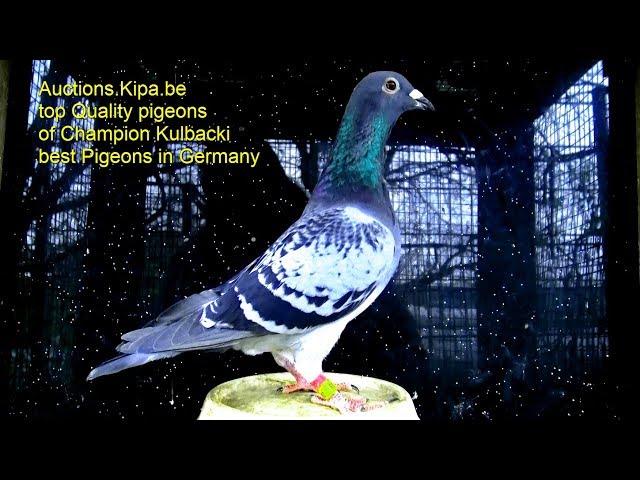The image is a digitally edited photograph of a pigeon, prominently centered and rendered in high detail. The pigeon stands upright on a greenish metallic, round surface, possibly a bowl. It exhibits vibrant blue feathers around its neck and head, with black feathers trimming its white wings and gray tail feathers. The bird's underside is white, complemented by its orange-colored feet with black claws and a green band around one of its legs.

The background gives an impression of being in a dimly lit, enclosed space, like a cage or aviary, with a surreal, heavily edited look that includes elements like stars and tree branches. The dark setting contrasts with the brightly lit pigeon, enhancing its visual prominence. Additionally, a snow-like pattern with white dots surrounds the pigeon, adding to the background's heavily edited feel.

Text in bright yellow is positioned in the upper left corner of the image, reading: "auctions.kipper.be. Top quality pigeons of champion Korbacke. Best pigeons in Germany." This suggests the image might serve as an advertisement or promotional material for selling high-quality pigeons.

Overall, the image blends a realistic portrayal of the pigeon with an almost otherworldly, edited backdrop, capturing focus on the bird and the promotional text.